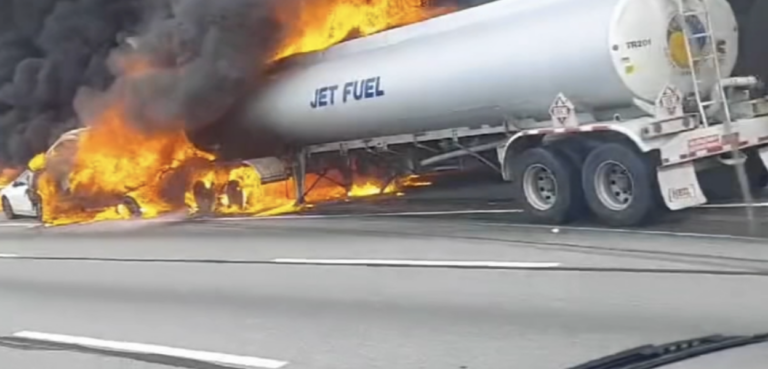The image captures a dramatic scene on a highway, taken from the vantage point of another vehicle's front window. The focus is a large silver tanker, labeled "JET FUEL" in navy blue letters, engulfed in intense orange and yellow flames. The front end of the tanker is completely consumed by fire, emitting plumes of thick black smoke into the sky. The tanker, resembling those towed by semi-trucks, features a metal ladder on its cylindrical body and has two sets of black wheels visible at the rear. In front of the burning tanker, the back end of a white vehicle is visible, also caught in the flames. The scene is brightly lit with natural daylight, highlighting the severity of the accident and the surrounding chaos on the highway.